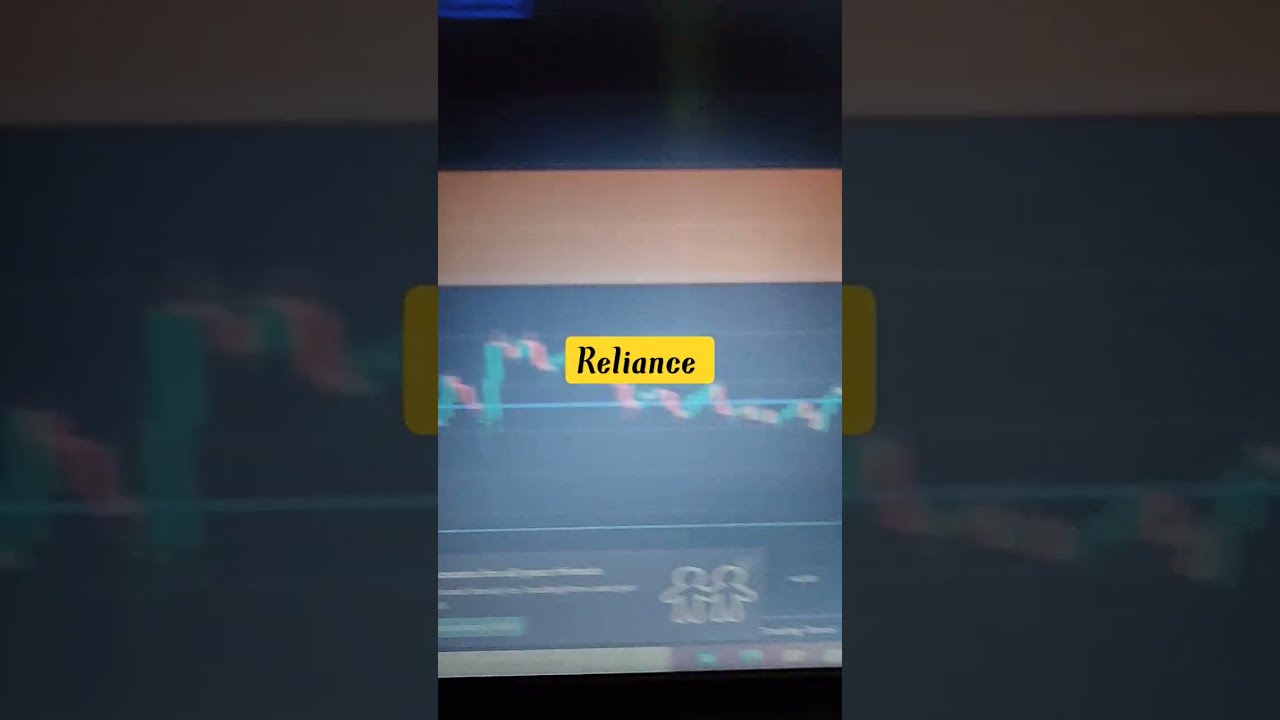The image depicts a layered composition with a picture within a picture. The inner photo is the main focus, appearing on a screen framed by a darker, zoomed-in version of the same image. The inner image's top third features a black background that appears to capture a photograph. Below this, a peach-colored bar transitions into a blue bar hosting a complex graph. The graph consists of overlapping thick lines in green and pink, resembling a heart rate monitor, running both horizontally and vertically across the monitor. Near the bottom of the image, there is another set of thin blue lines above a blurry gray box. Visibly outlined in white within this box are the silhouettes of two people, likely children, holding hands. Blurry white text appears next to the silhouettes, though it is unreadable due to the image's lack of focus. A prominent yellow box in the center bears the word “Reliance,” suggesting the image might illustrate a children's blackboard or a hospital monitor simulation. The entire scene is out of focus, lending the elements a dreamlike, indistinct quality.